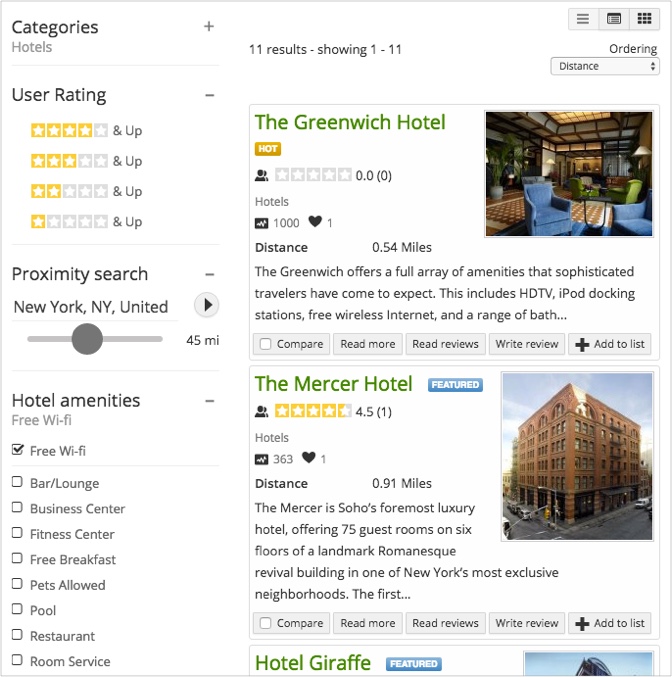The image displays a user interface for a hotel filtering system, characterized by a minimalist design and a light gray border in the upper left corner. At the top, the word "Categories" is written in a basic sans-serif gray font. Directly beneath it, "Hotels" is displayed in a smaller, lighter gray font, with a light gray divider line separating these sections.

Below the divider, the label "User Rating" appears in a bold black font, accompanied by a gray minus symbol to its right. A list of different star ratings follows, each with a descriptive text: "Four out of five and up", "Three out of five and up", "Two out of five and up", and "One out of five and up". Another light gray divider line is positioned underneath these ratings.

Continuing down, the section labeled "Proximity Search" is displayed in black font, with another gray minus symbol to the right. Beneath this heading, a smaller dark gray font reads "New York, NY, United..."—though the text is cut off. Adjacent to it is a gray circular icon with a darker gray border, featuring a dark blue play button in the center.

Following another divider line, there is a scrollable dark gray circle set against a light gray background line, representing a distance slider. To the right of the slider, "45 mi" is printed in small black font. Yet another light gray divider follows, leading to the "Hotel Amenities" section, noted in black font with a gray minus icon to its right.

Under "Hotel Amenities", the available options are listed in gray font, beginning with "Free Wi-Fi". A series of tick options are provided, with the selected option marked by a black check mark next to "Free Wi-Fi". The overall design is structured and clean, visually guiding the user through various filtering options for selecting a hotel.